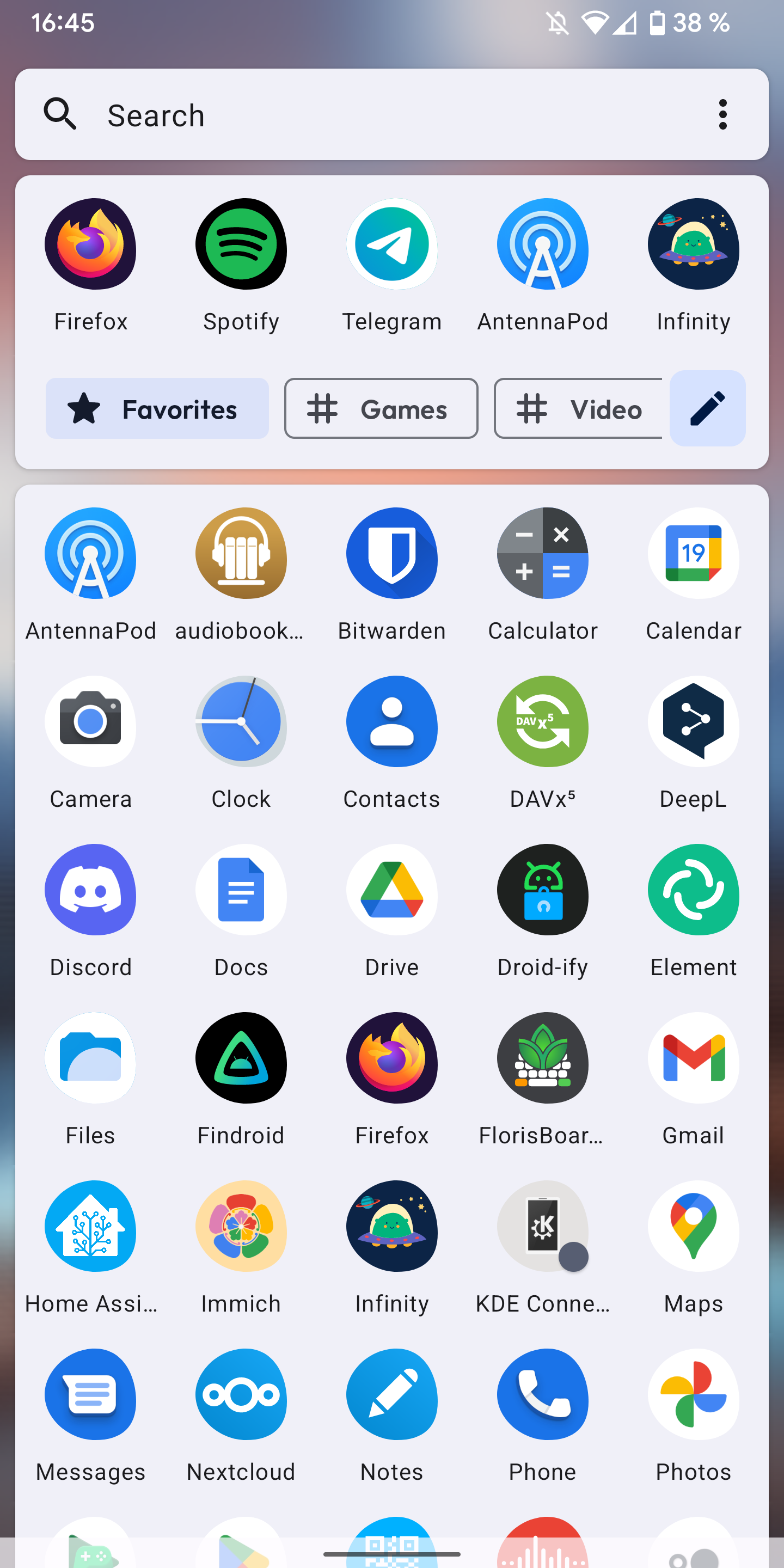This is a detailed screenshot of an individual's mobile phone home screen, showcasing a variety of apps. The device appears to be an Android phone, as indicated by the interface layout. The status bar at the top displays the time in military format as 16:45 on the left. The right side shows several icons: a silent mode symbol indicating notifications are muted, Wi-Fi connectivity, data signal strength, and a battery level at 38%.

Below the status bar, there is a search bar for easy access to quick searches. Directly underneath, the screen is segmented into 'priority apps' or 'favorites,' including Firefox, Spotify, Telegram, Antenapod, and Infinity. There are three navigational buttons below these apps labeled as 'Favorites,' 'Games,' and 'Video,' with 'Favorites' currently highlighted, suggesting the displayed apps are the user’s preferred choices.

The main app grid follows, filled with a multitude of applications—about 35 are visible. Noteworthy apps include Antenapod, Drive, Docs, Discord, Files, Fingeroid, Firefox, Gmail, Maps, Infinity, Messages, Notes, Phone, Photos, Calendar, and Calculator, arranged without a specific order.

At the bottom of the screen, a semi-transparent rectangular bar is faintly visible, which can be swiped up to access recent or currently open apps.

This screen provides a broad overview of the user’s app usage, indicating a diverse range of interests and functionalities.